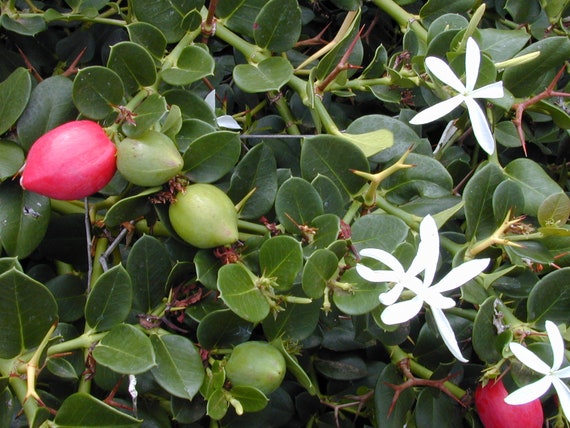The image captures a close-up view of a lush plant teeming with life, observed outdoors during the day. Centralized amidst greenery, the plant features numerous medium-sized, thick, and shiny leaves that are a rich green. The leaves are somewhat circular and stubby, with a small spike at their tips, growing off light green stems that have fine red-tinted thorns. These thorns, potentially acting as deterrents for birds and other fruit-eating animals, contrast against the delicate elements of the plant.

Scattered among the foliage are clusters of white flowers with long petals, each composed of five petals. Notably, three such flowers are grouped together near the bottom right, while a singular flower stands tall at the very top. The plant's stems also potentially carry flower buds, forming a vivid detail on the left side of the photograph, where three clusters can be seen, with one being red and the others green.

Adding to the plant's dynamic nature, various berries or fruits are found throughout: some still green and not yet ripened, while others showcase a vibrant red. These fruits are circular but end in a slight point, reminiscent of a rounded mango or a three-dimensional teardrop. The bottom right section of the image prominently features one red fruit, while additional red and green fruits are dispersed on the far left. The intricate details captured in this image reveal a thriving, multifaceted plant, intricately designed both to flourish and protect itself.